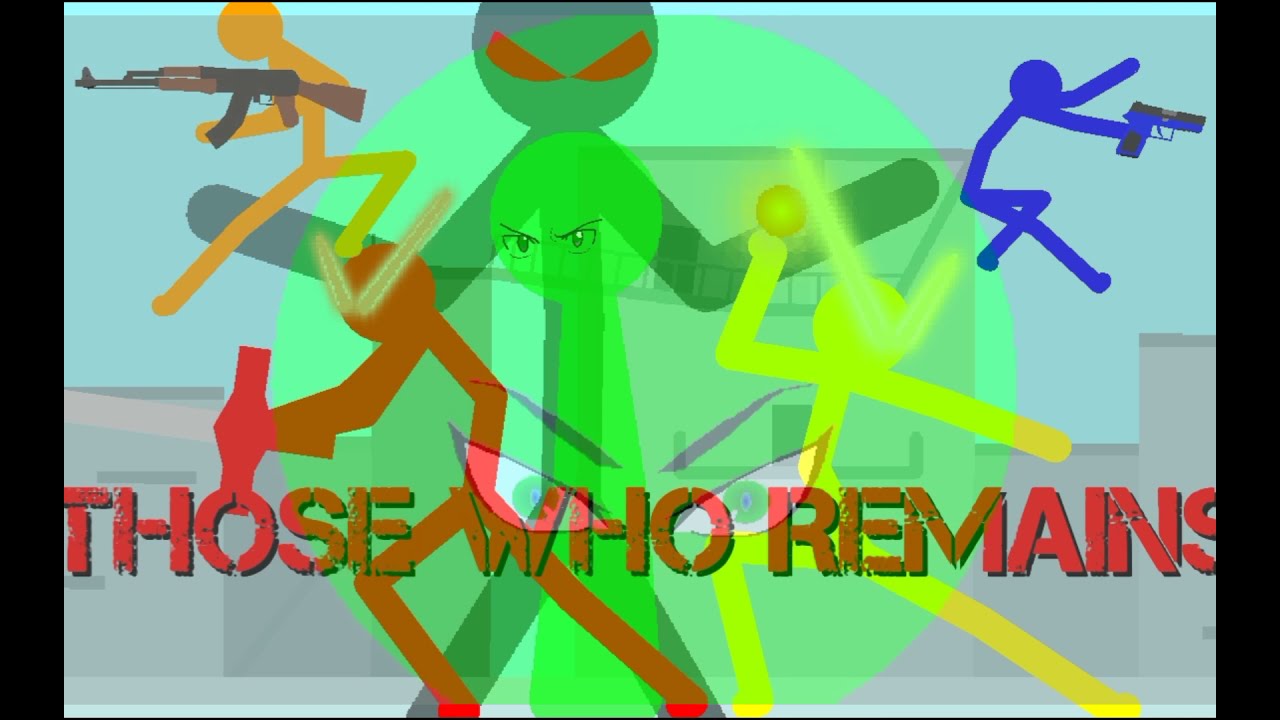The image is a slightly rectangular screenshot with thin black borders, depicting a scene from the beginning of a video game titled "Those Who Remain." It features several rudimentary, multicolored stick figures in dynamic, action-oriented poses. The figures are blue, orange, red, yellow, and two shades of green. Each stick figure is armed with different weapons: one with a 9mm pistol, another wielding a sledgehammer, one appears to be throwing an orange fireball, and another is holding an AK-47. In the center is a large lime green stick figure with red eyes and outstretched arms, standing in front of a transparent green circle. The background includes abstract detailing, such as a bridge, a keyhole with eyes peering through, and yellow lines at the bottom. Red text at the bottom of the image declares the game title, "Those Who Remain." The chaotic and hyperactive nature of the figures, along with their weaponry, suggests a sense of violent urgency.